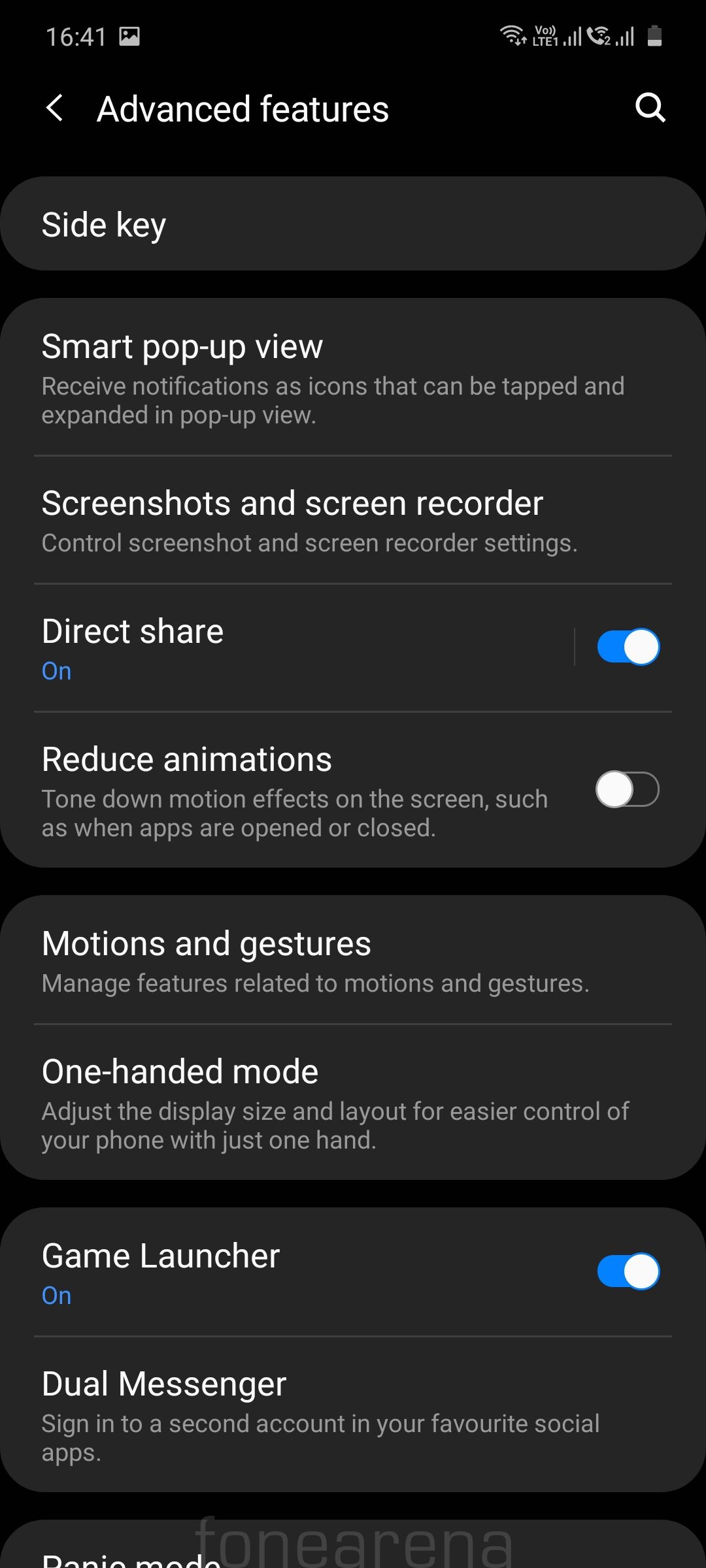**Detailed Caption:**

A screenshot of a smartphone's settings interface, showcasing various advanced features and options. The device is connected to the "1641 Gallery" Wi-Fi network, indicated by full bars, and also has full signal strength for voice calls with a Wi-Fi Phone 2 connection. The battery level is at approximately 25%.

The settings menu displays key features including:

- **Arrow Back:** An option to navigate back to the previous screen.
- **Search Function:** To easily find specific settings or features.
- **Side Key:** Configurations for the physical side buttons on the phone.
- **Smart Pop-up View:** Enables notifications to appear as icons that can be tapped and expanded into pop-up views.
- **Screenshots and Screen Recorder:** Control settings for capturing and recording screen activity.
- **Direct Share:** An active feature for quickly sharing content with frequently used contacts or apps.
- **Reduce Animations:** A toggleable option to minimize motion effects when opening or closing apps, currently turned off.
- **Motions and Gestures:** Settings to manage features related to physical motions and gestures.
- **One-handed Mode:** Adjust display size and layout for easier phone control with one hand.
- **Game Launcher:** Enabled for an optimized gaming experience.
- **Dual Messenger:** Allows signing into a second account in social media apps.

Overall, the image provides a comprehensive view of the phone’s customization and accessibility options to enhance user experience.